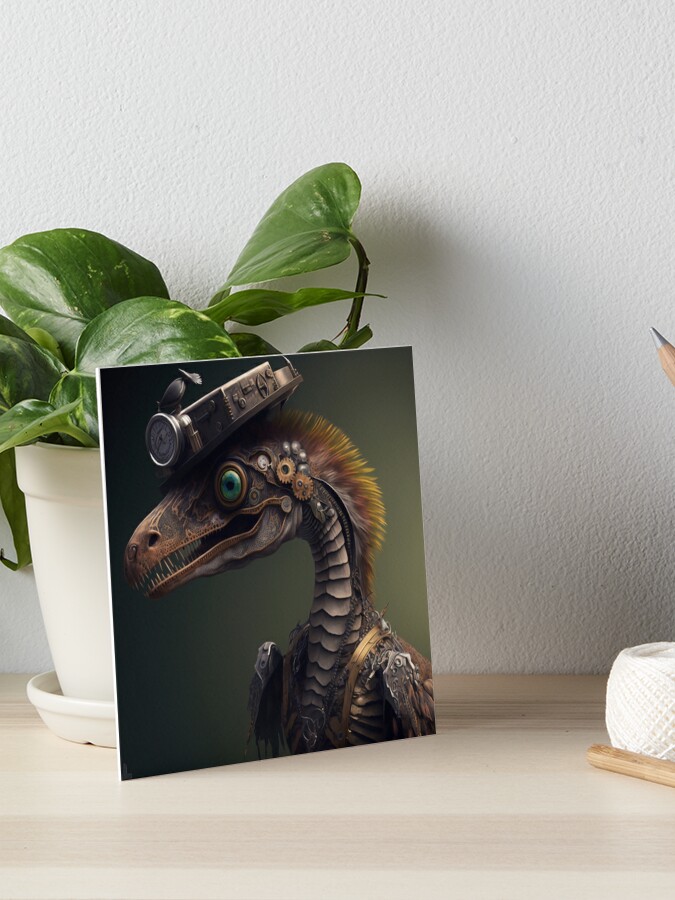On a whitewashed natural wooden shelf against a light-colored wall, a charming scene unfolds. Dominating the shelf is a white planter with a matching dish beneath, holding a lush plant whose big, slightly variegated, heart-shaped leaves stretch out. Propped up against the planter, a striking artistic rendering captures attention: it features a fantastical creature with the snout of a dinosaur adorned with a really large blue eye, sharp teeth, and intricate mechanical parts including a yellow mohawk and a headpiece resembling a compass or camera. The creature's neck is embellished with large scales, enhancing its otherworldly appearance. To the right of this intriguing artwork is a small white porcelain object, possibly a dish or vase, with a wooden item in front of it. Above this wooden object, the silver tip of a pencil peeks out, adding an extra element of curiosity to the carefully composed shelf display.